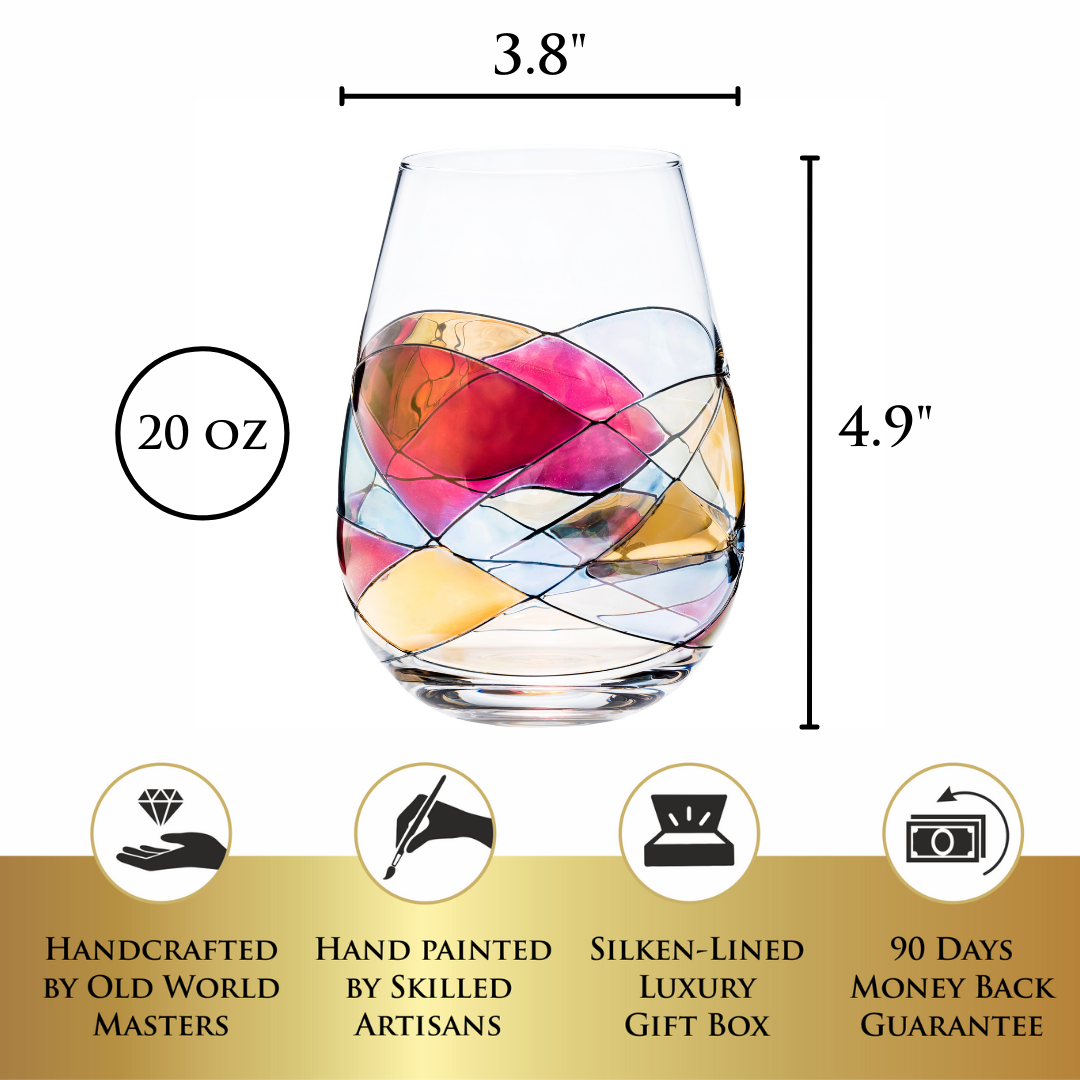This is a photograph of a clear glass tumbler, adorned with a stained glass-like pattern featuring a colorful mosaic of ovals in yellow, red, pink, light blue, brown, gold, and orange. The glass narrows at the top and widens at the bottom, with dimensions displayed on the image: 20 ounces capacity is indicated in a black circle on the left, 3.8 inches in width marked at the top, and 4.9 inches in height marked on the right. A gold metallic strip at the bottom carries black text and icons: it reads "handcrafted by old world masters" with an adjacent icon of a black hand holding a diamond, "hand-painted by skilled artisans" with an icon of a hand with a paintbrush, "silken lined luxury gift box" accompanied by an image of a gift box, and "90 days money-back guarantee" with an icon of currency encircled by an arrow. The entire arrangement is set against a white background.